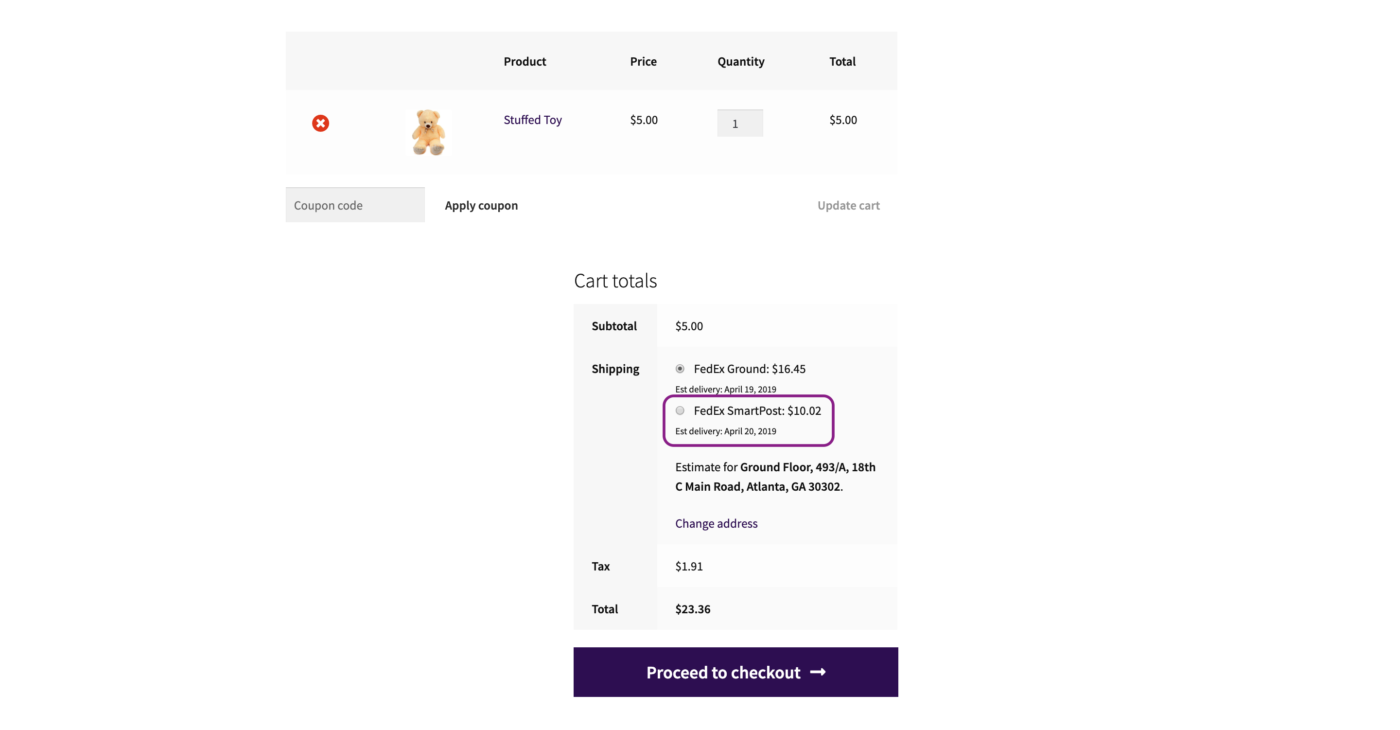The image captures the view from within a shopping cart interface on an e-commerce website. Dominating the top right, four categories are displayed from right to left: "Total," "Quantity," "Price," and "Product." In the "Total" column, a value of "$5" is noted, while under "Quantity," a small box containing the number "1" is visible. Adjacent to this, the "Price" column lists an amount of "$5," and the "Product" column describes the item as a "Stuffed Toy."

Further left, an image showcases the actual product, which appears to be a light brown stuffed bear toy. To the left of this image is an "X" icon, potentially for removing the item from the cart. Beneath the product image, a box labeled "Coupon Code" invites users to enter a discount code, with an "Apply Coupon" button situated to its right. 

Further down the interface, the right side highlights an "Update Cart" option under the "Total" column. At the bottom right, encased in a squared-off section titled "Cart Totals," the breakdown includes a "Subtotal" of "$5," alongside placeholders for "Shipping" and "Tax," culminating in the final "Total." Lastly, a prominent purple box at the bottom right encourages users to "Proceed to Checkout," marked by a white arrow pointing to the right.